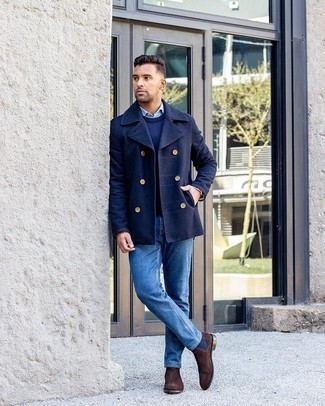A stylishly dressed man is depicted in this outdoor fashion shot, leaning casually against a white stone building that features tall glass doors with a light brown frame and a window above. The man, who has a well-trimmed short beard and neatly styled short black hair—longer on top with shaved sides—is wearing a dark blue, double-breasted jacket with six wooden buttons, blue jeans, and dark brown Chelsea boots. His pose is relaxed but deliberate: one hand in his pocket, the other hanging by his side, his left leg straight, and his right leg bent and crossed lightly in front of it with the toe resting on the ground. He gazes thoughtfully to his right. Through the glass, a two-story building with railings and a tree are visible, adding depth to the scene. The area around him is paved with concrete. No other people or text are present, emphasizing the man's fashionable presence against the minimalist backdrop.